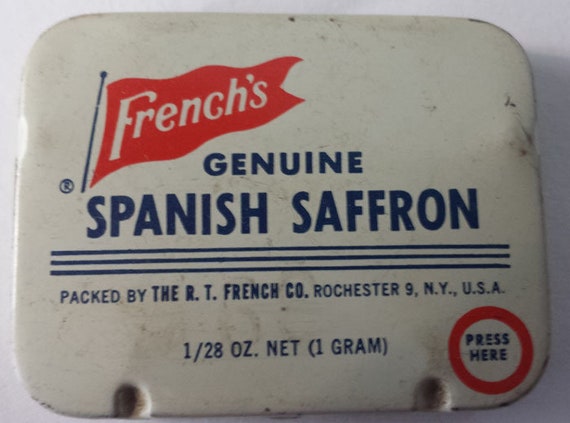A close-up indoor photograph captures an old, slightly scratched, and dirty white tin container lid. Prominently positioned in the upper left corner, there is a red flag logo with the brand name "French's" written in white. Below the flag, in bold navy blue capital letters, it says "Genuine Spanish Saffron." This text is followed by three horizontal blue lines. Further down, in smaller blue print, it reads "Packed by the R.T. French Co., Rochester 9, NY, USA." Below this, the text indicates the weight as "1/28 ounce, net 1 gram" in blue characters. On the right side of the lid, there's a red circle with a white center that instructs "Press Here" in blue letters. The overall condition of the container suggests it is quite old and has seen considerable use, as indicated by the various scuffs and marks on its surface.